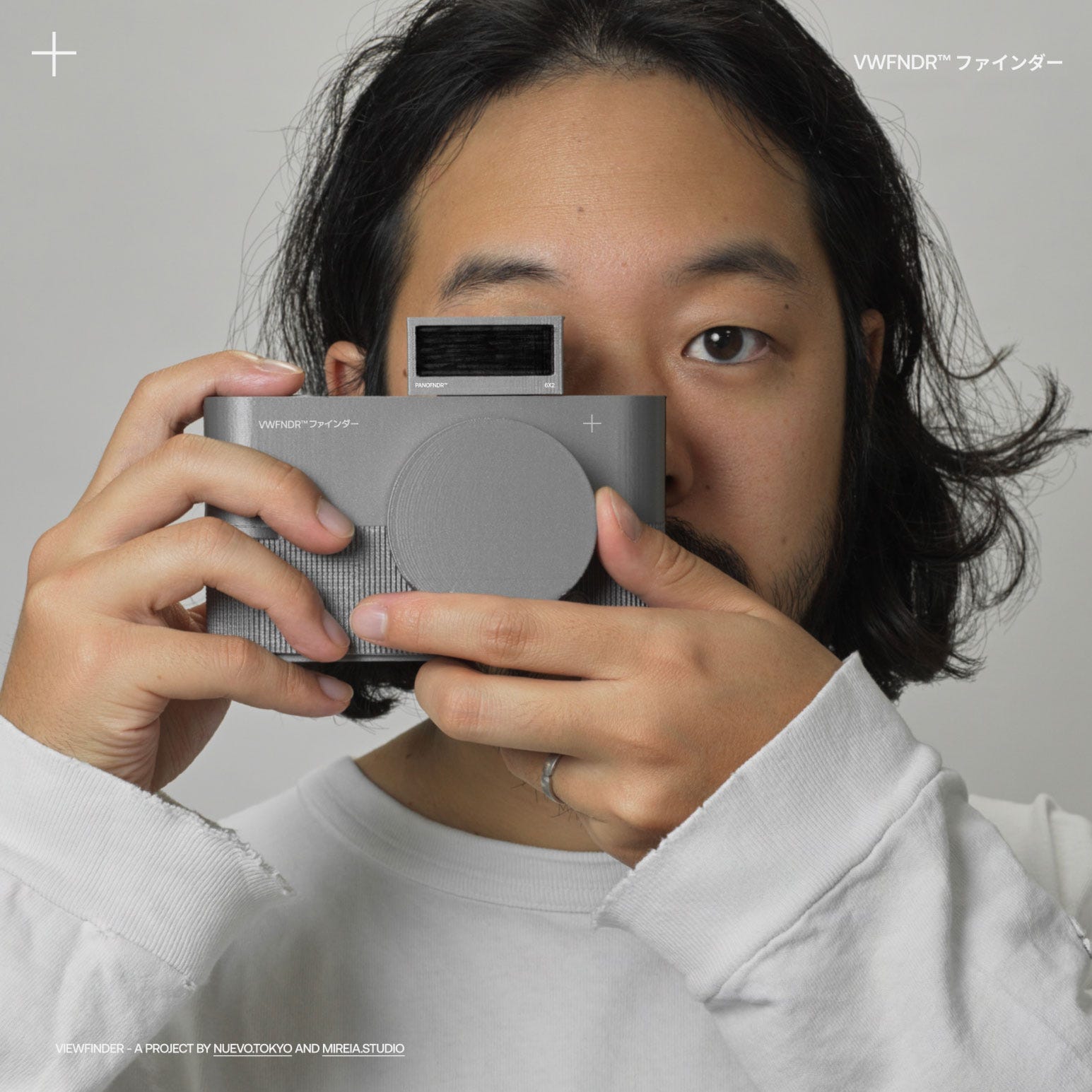The image features a close-up view from the shoulders up of an Asian man, approximately 30 years old, with dark hair that falls past his ears. He is wearing a white, long-sleeved shirt, with frayed edges at the cuffs, and a silver wedding band on his ring finger. The man is holding a futuristic grey camera labeled "VW Finder" and is looking directly at the viewer, with one eye on the viewfinder of the camera. The background is a light grey, suggesting it could be part of an advertisement. In the top right corner, there is the "VW FNDR" trademark alongside some letters in an Asian language. Additionally, a white plus sign is visible in the top left corner. At the bottom left of the image, there are small letters that read, "VW FNDR, a project by Nuevo.Tokyo and Miera.Studio."